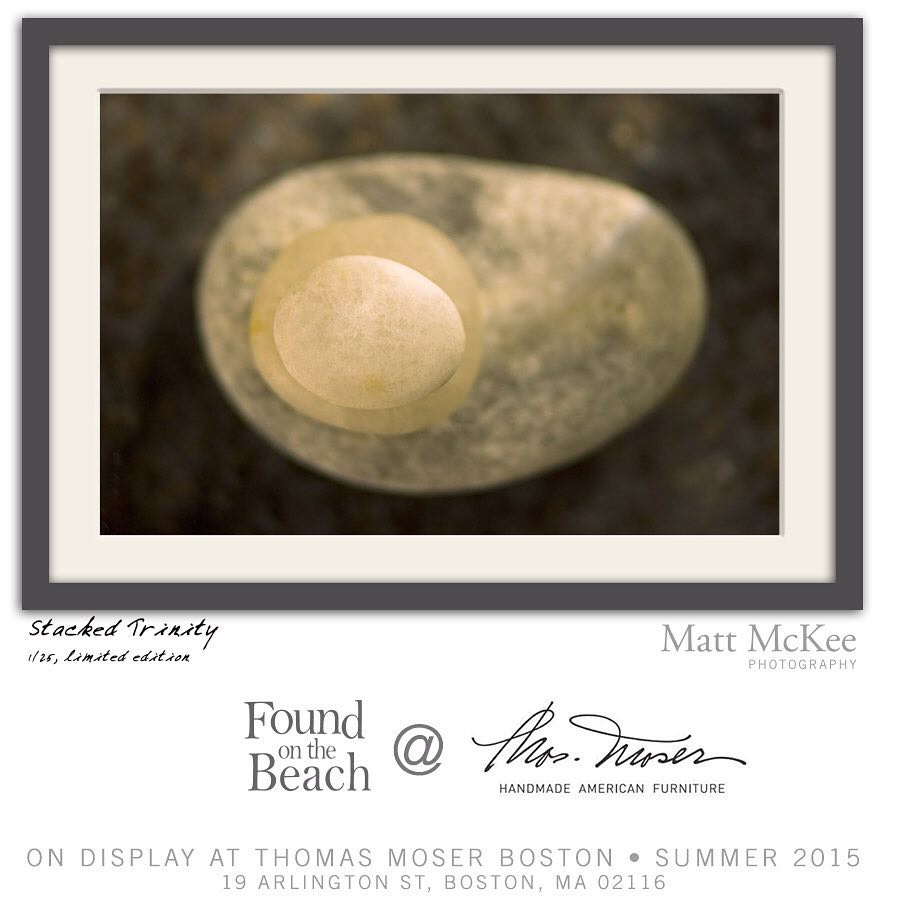The image is a matted photograph framed with a gray bordered rectangular frame and white matting. At the center of this frame is a slightly blurry close-up of what appears to be three white stones stacked on top of each other, resembling an egg in a pan. This stone arrangement is presented against a dark background. Below the image, there is an inscription in small black cursive font that reads "Stacked Trinity 125 Limited Edition" on the left, and "Matt McKee Photography" on the right. Further below, centrally aligned, it states "Found on the Beach" and appears to be followed by an indistinct handwritten name, possibly related to "Handmade American Furniture." At the very bottom, it reads "On Display at Thomas Moser, Boston, Summer 2015," and then provides the address, "19 Arlington Street, Boston, MA 02116." This descriptive caption gives details about the visual elements of the photograph and its framing, as well as exhibition details, suggesting it may be part of an art show or gallery display.